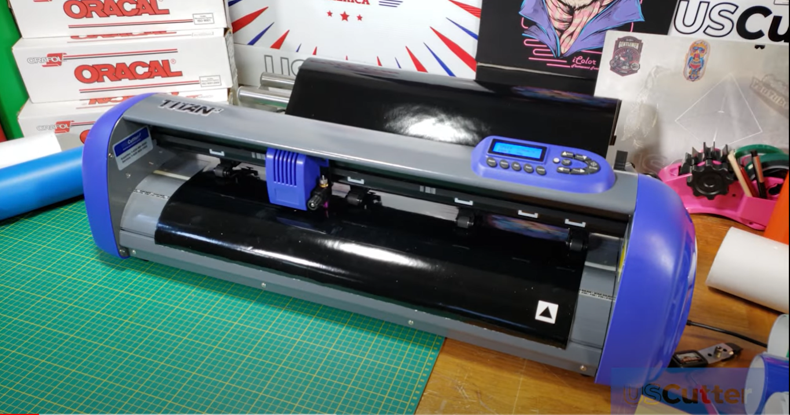This is a detailed photograph of a long, blue and gray instrument, resembling a printer or cutter, with a transparent front panel and a prominent black roller section. The instrument, marked with the brand name "Titan" and featuring buttons on its top right, sits on a light wood craft table. To the right of the instrument is a green, self-healing cutting mat with a grid pattern. In the background, a collection of white boxes labeled "ORACAL" can be seen, alongside additional crafting supplies like paper rolls and tools. The scene captures an organized workspace with personal artwork on display in the upper right corner, suggesting a creative environment tailored for crafting projects.